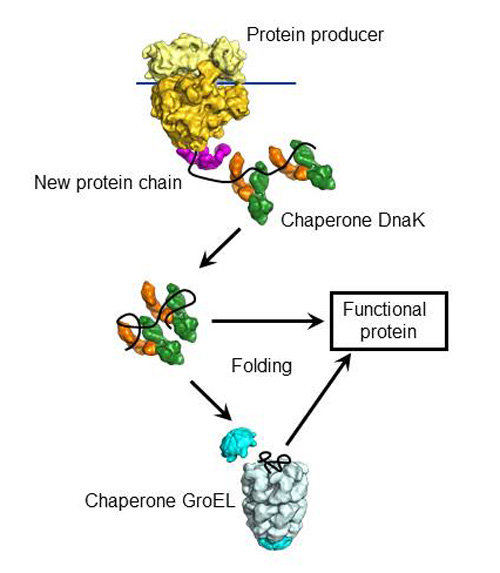The image depicts a detailed diagram illustrating the process of protein production. At the top, there is a complex, wrinkly structure reminiscent of a piece of ginger, colored predominantly in light beige at the top, transitioning to a ginger hue in the middle and purple at the bottom. This structure is labeled "Protein Producer" and resembles the shape of either a bunch of grapes or South America.

Emerging from the Protein Producer is a black line adorned with orange and green globs, labeled "New Protein Chain." An arrow points from this new protein chain towards the right where it leads to a mass labeled "Chaperone DNAK," colored in green and orange. 

From the Chaperone DNAK, another arrow directs the flow towards a square labeled "Functional Protein," signifying the newly formed protein's functional state. Additionally, an arrow moves upward from this green and orange mass towards the Functional Protein, implying a folding process. 

Another arrow extends downward from the new protein chain towards a blue, floating glob and another mass composed of what appear to be white stones at the top and blue at the bottom, labeled "Chaperone GROEL." This blue mass signifies an alternative pathway or additional folding step with the aid of the GROEL chaperone.

In summary, this visual guide traces the journey from a Protein Producer through intermediate stages involving chaperones DNAK and GROEL towards the formation of properly folded and functional proteins, capturing the intricate and sequential nature of protein synthesis and folding.